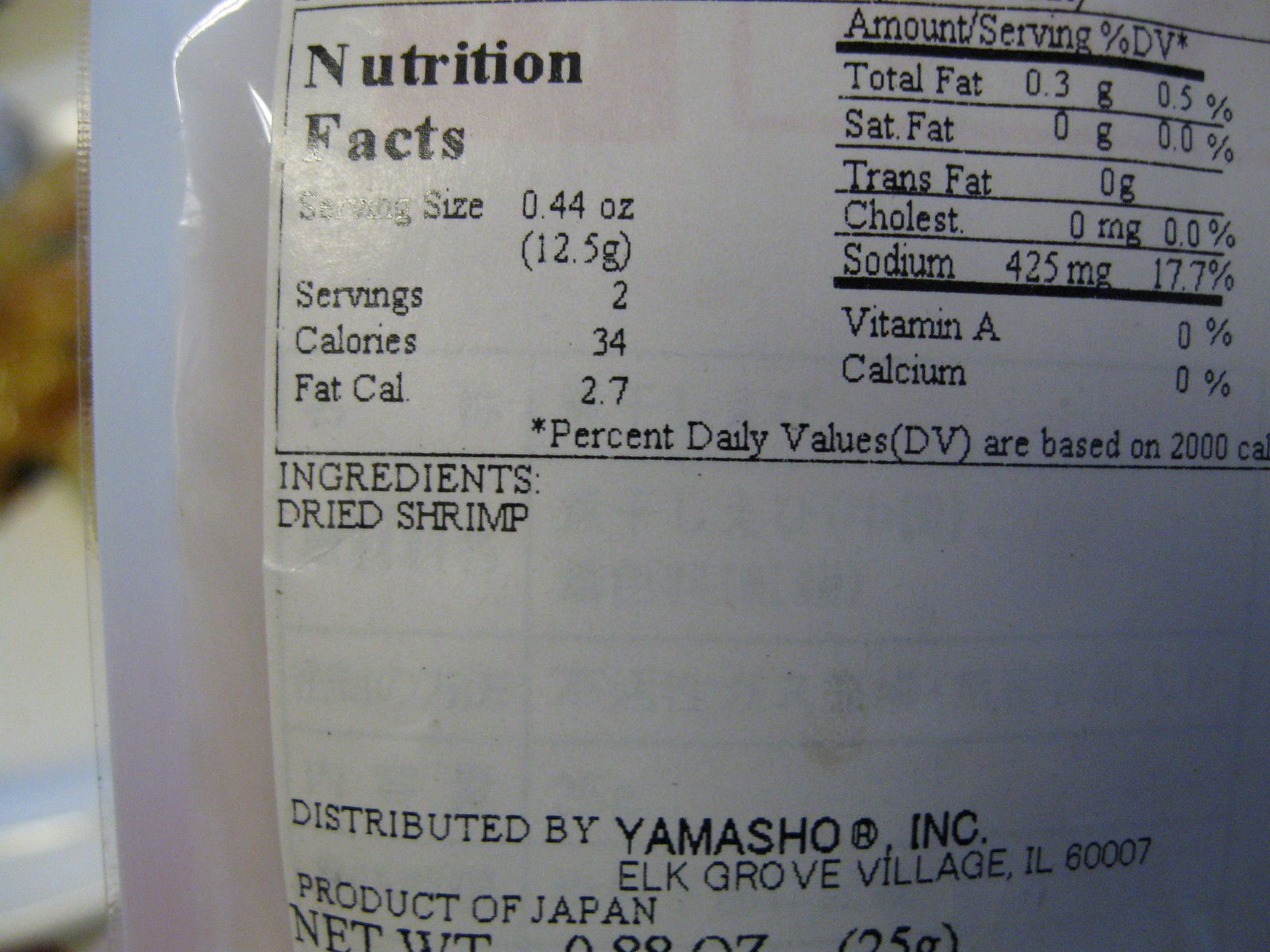A detailed caption for the image:

"This image showcases a detailed nutrition label for a Japanese product, including vital information such as serving size, caloric content, and amounts of fat and salt. Below the nutrition facts, the label lists ingredients, including dry shrimp. The product is distributed by Yamashu Incorporated, based in Elk Grove Village, Illinois (ZIP code 60007), and is manufactured in Japan. The nutrition label is printed in black and white on standard white paper, which is enclosed in a transparent, laminated covering, ensuring durability and protection."